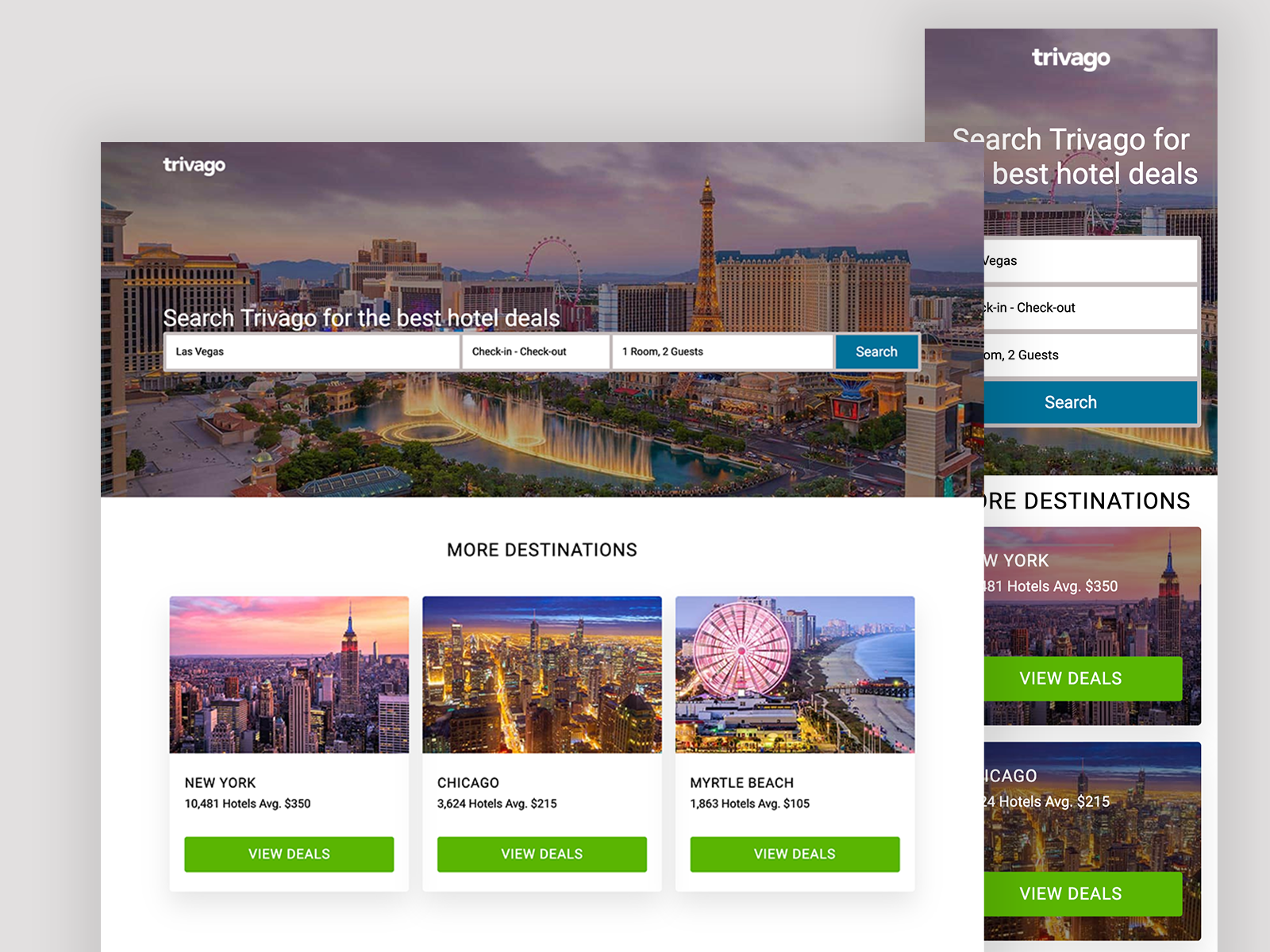The image depicts a screenshot of the Trivago website. At the top, there's a search bar with fields for the destination, check-in and check-out dates, the number of rooms, and the number of guests, currently set to Las Vegas, with a search button highlighted in blue. Below, there are sections highlighting hotel deals in various cities.

The background features an image of New York City, showing the iconic skyline with prices indicating hotels averaging $3.50.

To the right, a green rectangle is labeled "Videos," with corresponding details for Chicago, where hotels average $2.50. The Chicago section features a striking image of the cityscape with brightly lit skyscrapers, bridges, and cars.

Further down, there's information on Myrtle Beach, which includes a visual of a Ferris wheel, water on the right, sand, and a pier, all illuminated against a dark backdrop.

Other cities such as New York and Las Vegas have their own specific blocks, with New York's hotel prices averaging around $15, and Chicago showing another statistic of $215 average. The Myrtle Beach section indicates another entry, featuring specific nighttime attractions.

Overall, the image serves as a comprehensive demonstration of how the Trivago interface organizes and presents hotel deal information, highlighting key destinations with vivid imagery and pricing details.